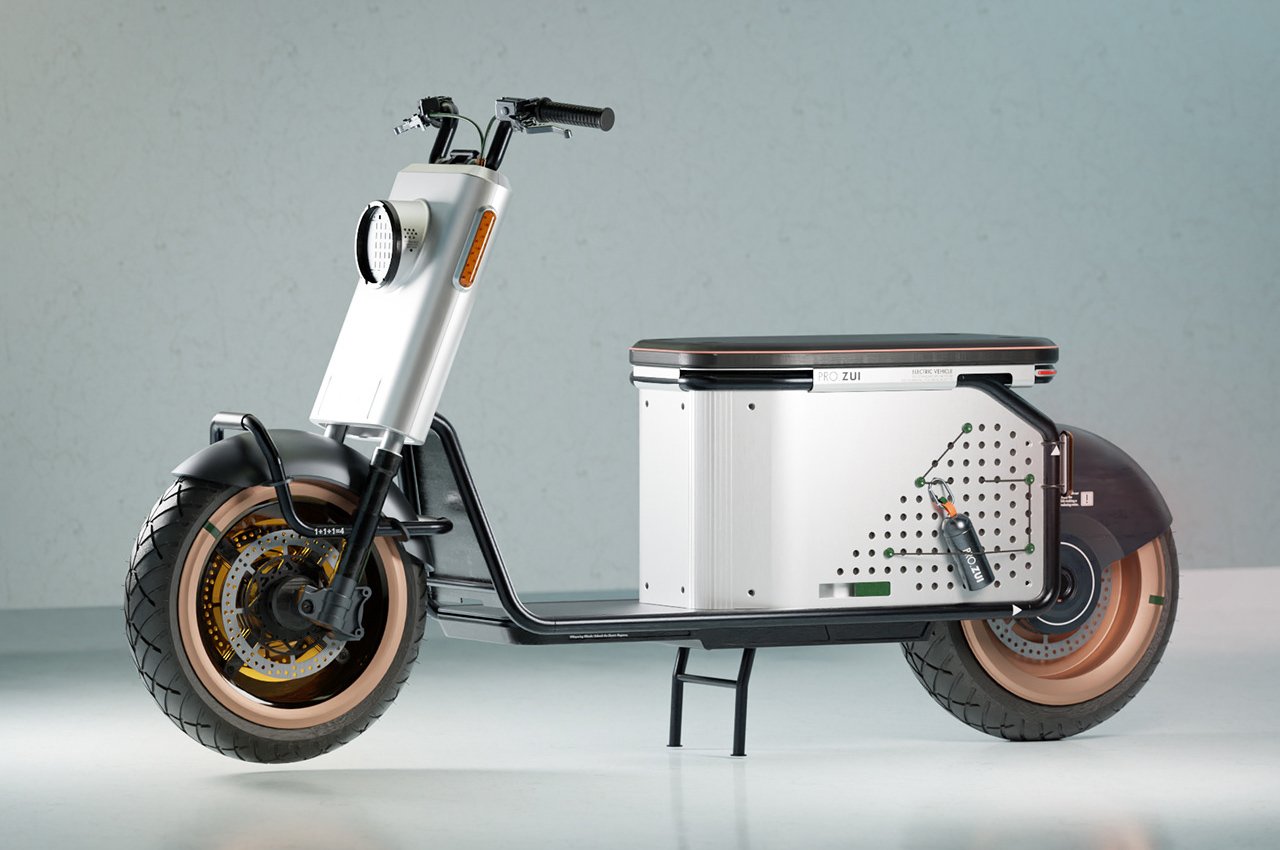The image is a pristine, computer-generated or AI-created depiction of a sleek, white and silver motorbike resembling a cross between a bicycle and a scooter. The bike, facing towards the left, is set on a reflective white floor with a plain gray background, enhancing its modern, almost futuristic aesthetic. It features chrome rims on both its large black tires and is balanced by a black kickstand underneath. The handlebars are black, and a headlight adorns the front of the bike. Below the seat, there appears to be a white box, likely for storage or possibly housing an electrical component, suggesting the bike is electric as there is no visible gas tank. The brand name "Prozui" (P-R-O-Z-U-I) is prominently displayed, although other text on the bike is minimal and inconspicuous.